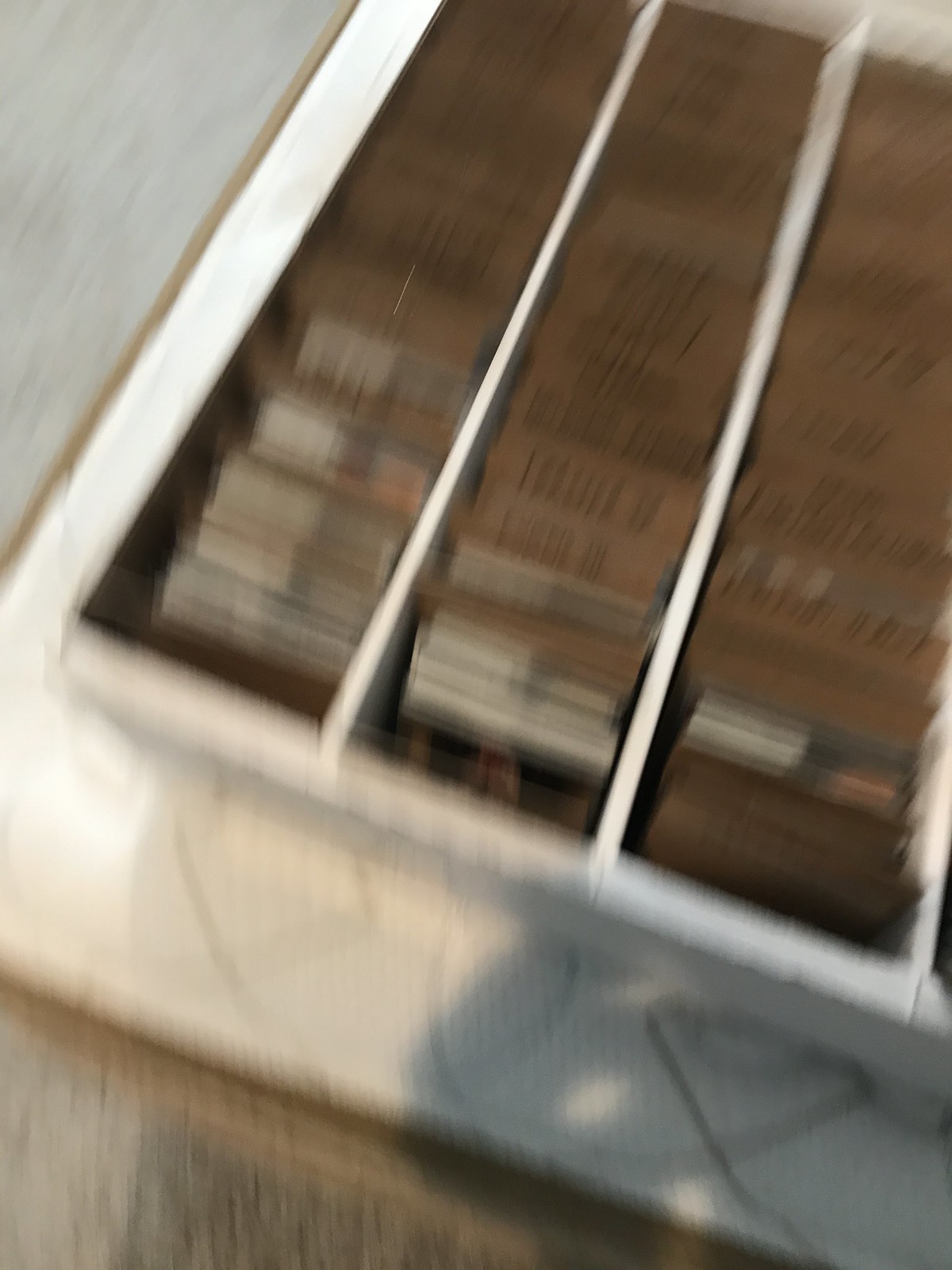This photograph depicts a small, card-catalog-style filing system situated in a brightly lit room. Though the image is extremely blurry, three distinct rows are visible, resembling a compact file system typically used for organizing items such as baseball cards. The structure encasing these rows is white, providing a stark contrast against the blurred details. Each row appears to have dividers—likely made of brown material—interspersed throughout, with what seems to be illegible writing marking each section. Notably, in the foreground of the image, the shadow of the person taking the photograph is prominently cast, adding a human element to this otherwise unclear snapshot.